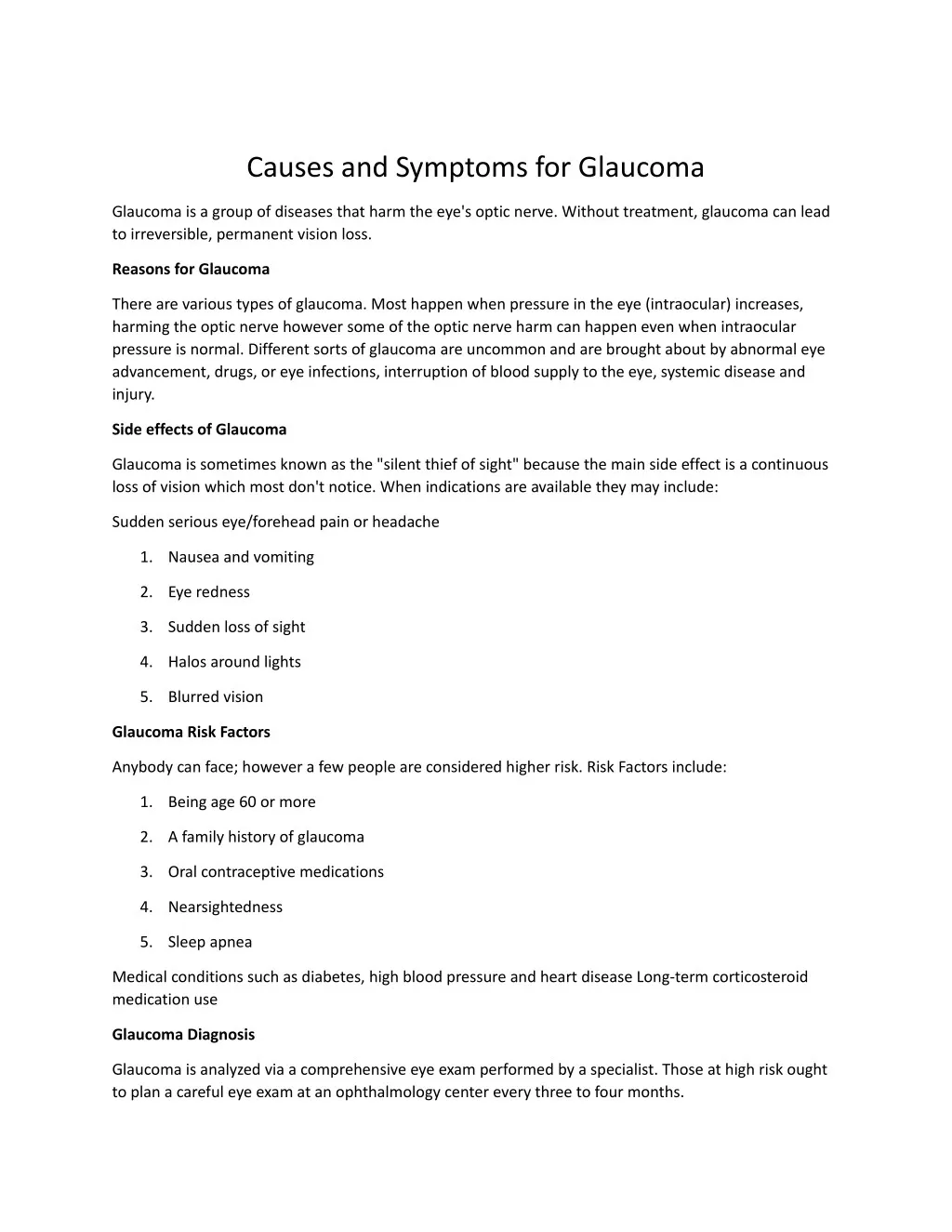### Detailed Caption for an Image

The image appears to be a screenshot of a web page titled "Causes and Symptoms for Glaucoma," presented on a completely white background with black text. 

The content begins by explaining that glaucoma is a group of diseases that damage the eye's optic nerve. It warns that, without treatment, glaucoma can lead to irreversible and permanent vision loss.

The next section, titled "Reasons for Glaucoma," states that there are several types of glaucoma, most of which occur when the pressure inside the eye increases, harming the optic nerve. However, it also notes that optic nerve damage can happen even when intraocular pressure is normal. Other, less common causes of glaucoma are attributed to abnormal eye development, certain medications, eye infections, disruptions in the blood supply to the eye, systemic diseases, and injuries.

Further down the page is a section on the "Side Effects of Glaucoma." This part lists symptoms such as sudden, severe eye or forehead pain, headaches, nausea and vomiting, redness in the eye, sudden loss of sight, seeing halos around lights, and blurred vision.

The page concludes with information on "Glaucoma Risk Factors," identifying age (60 or over), a family history of glaucoma, oral contraceptive medication, nearsightedness, and sleep apnea as contributing factors.